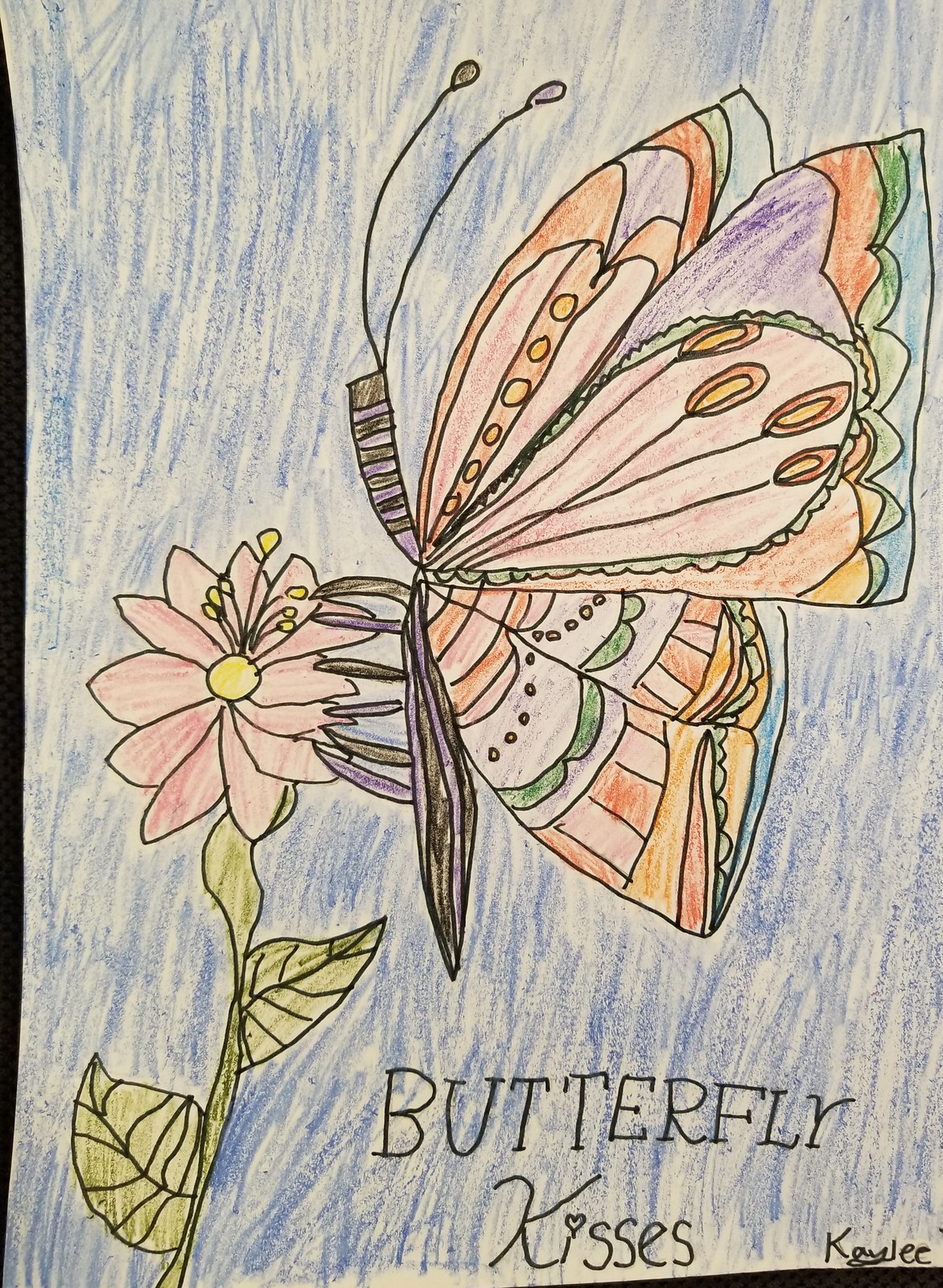This is a charming, hand-colored picture, likely created by a child. The background is filled with vibrant blue, reflecting an enthusiastic, albeit untamed, approach to coloring, as the strokes exceed the designated boundaries. In the bottom right corner, there is a pink flower with a myriad of petals surrounding a cheerful yellow center. The flower's light green leaves and stems emerge with a fresh, lively appearance. 

To the left, a beautifully detailed butterfly clings to the flower. The butterfly's body is segmented into a triangular lower portion and a rectangular upper part, complete with two delicate antennae. Its four wings are symmetrically colored in a delightful palette of oranges, greens, pinks, yellows, blues, and purples, showcasing the child’s careful attempt to emulate the natural patterns of a butterfly.

At the bottom left, the phrase "Butterfly KISSES" is inscribed, with "KISSES" notably capitalized except for the 'K.’ The artwork is signed by "Kaylee" in the lower left corner, adding a personal touch to this colorful, whimsical scene.